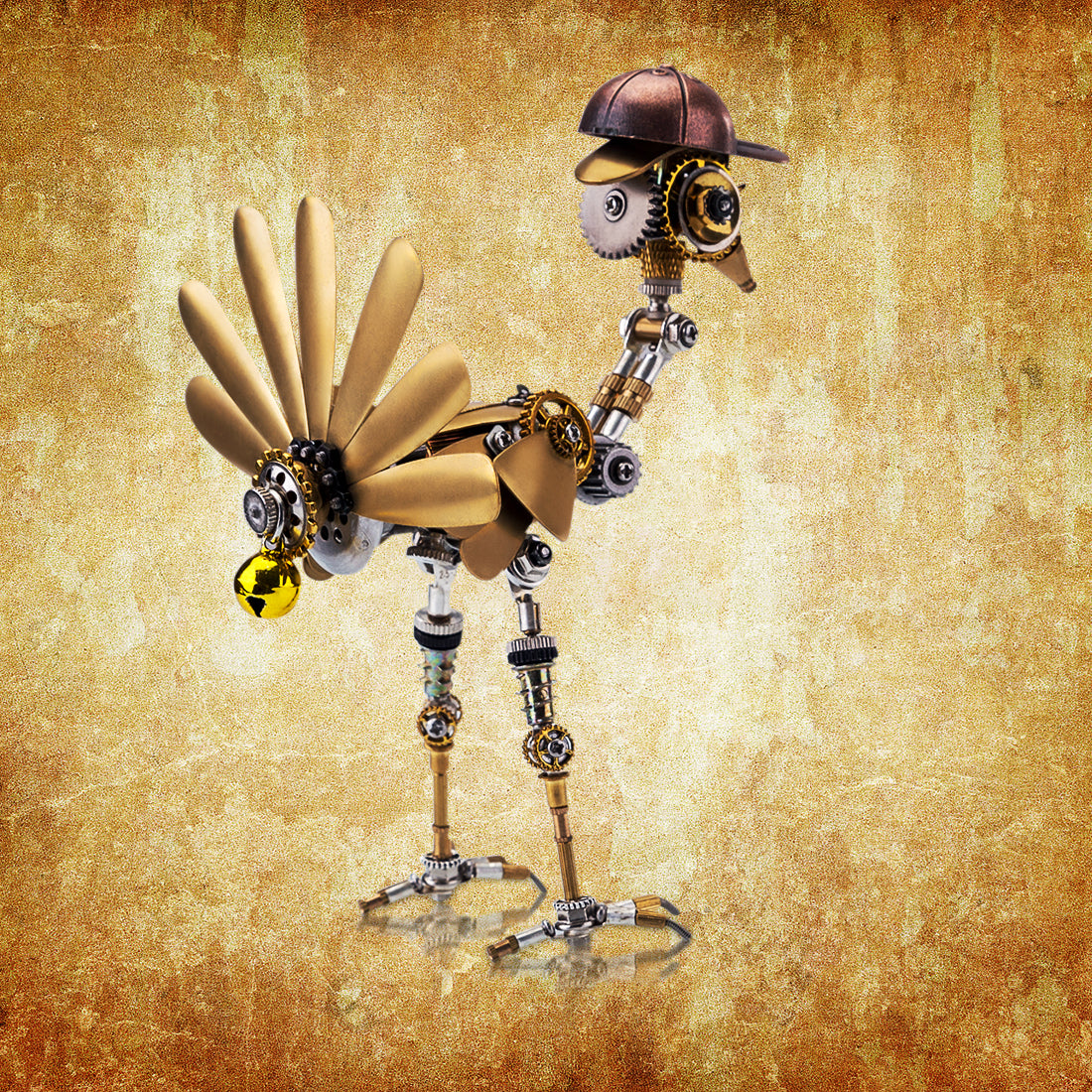In this intriguing image, we see an abstract, steampunk-inspired depiction of a mechanized bird, viewed from a back-side angle. The bird's body is a complex collage of various mechanical parts, giving it a distinctly robotic appearance. Its tail resembles a set of golden fan blades, divided into six distinct sections, each detailed with intricate robotic mechanisms. The wings, also fan-like, add to its mechanical aesthetic. The bird's head, adorned with gears and a funnel-shaped piece of metal, sports a red metallic baseball cap, contributing to its quirky charm. A small yellow orb, reminiscent of a Christmas ornament, hangs off the very back of the creature, adding a whimsical touch. The background of the image is predominantly a rich, streaky gold-bronze texture, with a lighter patch in the center, providing a contrasting backdrop that highlights the mechanical intricacies of the bird-like figure.